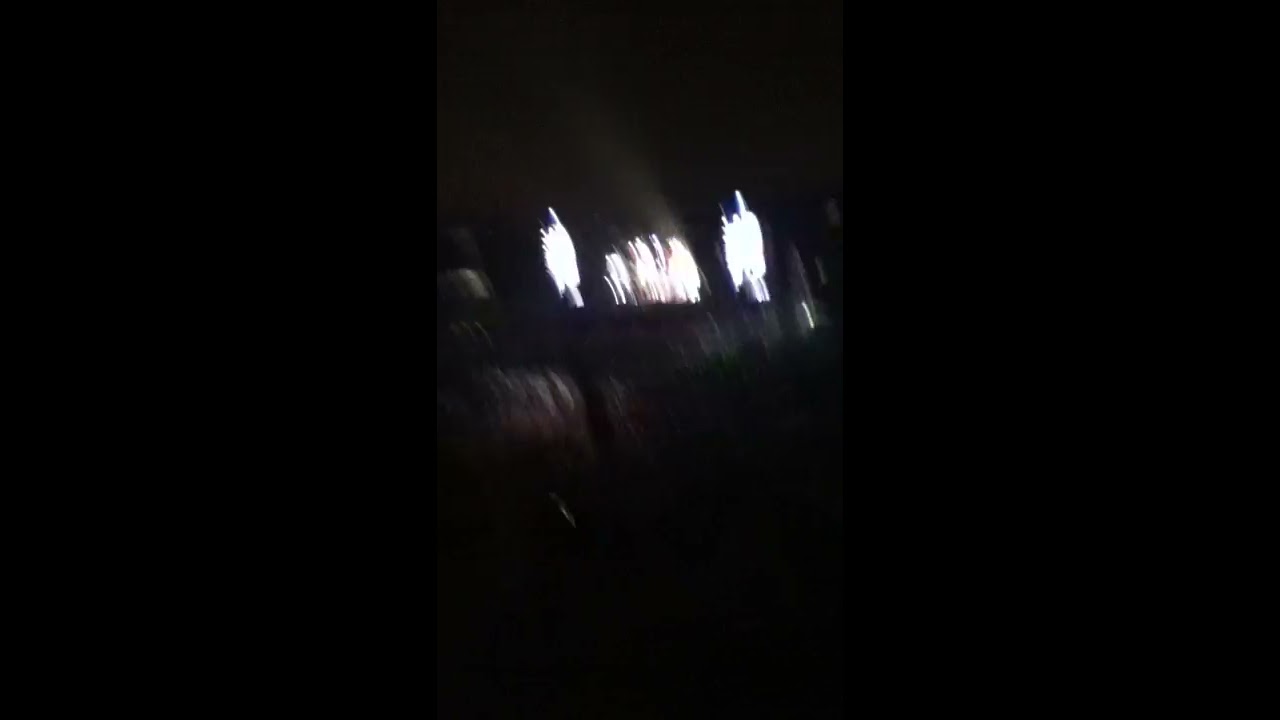This image is a horizontally aligned rectangular photograph, framed by thick vertical black borders on both the left and right sides, creating a narrow central viewing area. The predominant color in the image is black, with very little detail visible due to extreme blurriness. At the top, a black expanse is interrupted by a small streak of white. Below this, several bright white shapes emerge, appearing as indistinct and scraggly forms—possibly due to camera movement—resembling elongated squiggly lines or scribbles. These streaks, numbering around five, seem to vibrate up and down. Towards the middle and bottom sections, the white streaks become fainter and blend with grayish, smoky, and blurry areas before the image transitions back to solid black at the very bottom. The white, blurry objects are the primary focal point, although they are indistinguishable and lack clear definition, making the overall scene almost indecipherable.